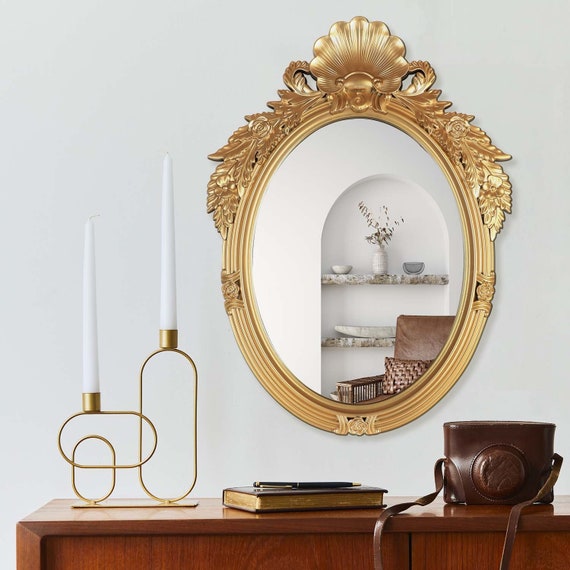This color photograph captures a detailed interior scene featuring a white wall adorned with an elaborate gold-framed mirror. The mirror, which boasts intricate designs of grape leaves, flowers, and a seashell motif on top, reflects a portion of the room opposite, revealing a brown leather chair with a matching pillow and a set of shelves. These shelves hold a flower pot, two bowls, and a large serving dish.

Beneath the mirror stands a medium brown wooden cabinet with sliding doors. Atop this cabinet lies a brown leather camera case with a long thin strap hanging over the edge, a brown leather-bound book with gold-edged pages, and a tall light fixture resembling candles set in wire frame bases shaped like oval racetracks. Additionally, a black pen rests on the book. The overall composition suggests careful placement and possibly digital manipulation, as no photographer is visible in the mirror's reflection.